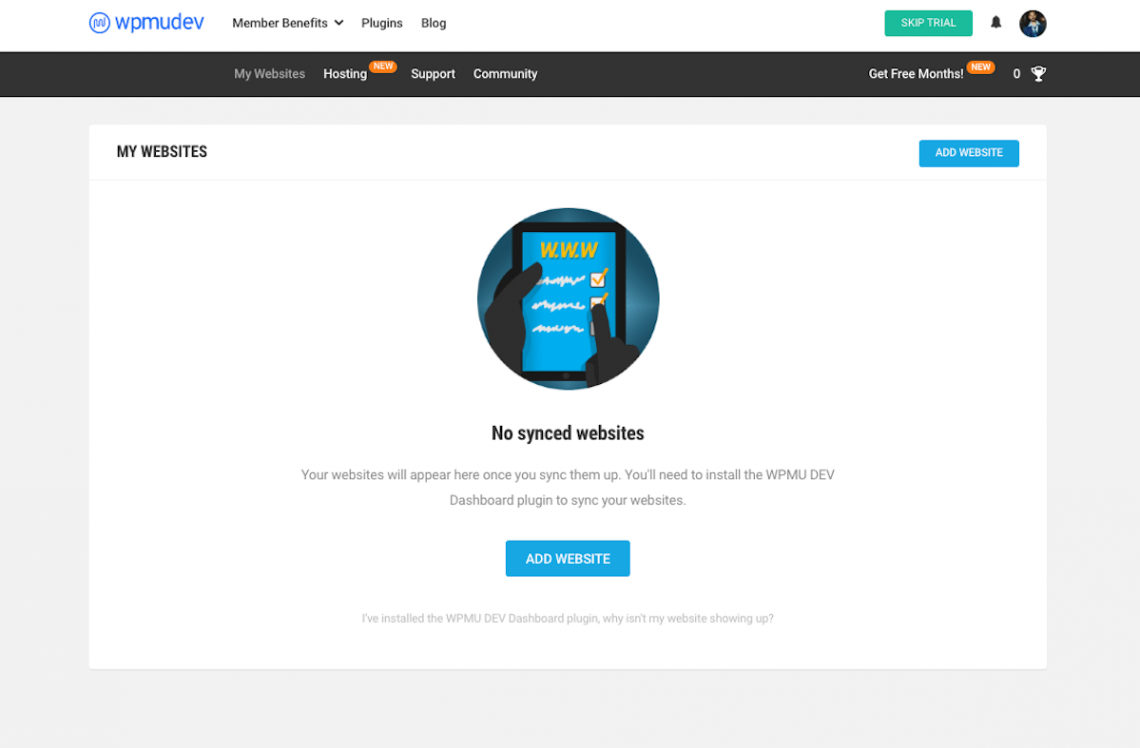At the top of the image, there's a blue header featuring a circle with a jagged line in the middle, and the text "Member Benefits Plug-in Blog." To the right of this header is a green button labeled "Skip Trial." Below this header, there is a black box with the text "My Website Hosting" written on it. Next to this text is an orange button marked "NEW." 

Underneath, there is a section that includes options such as "Support," "Community," and "Get Free Months." Another orange button labeled "NEW" is also present in this section, along with a trophy icon.

Further down, there's a light gray area that contains a large white rectangle. On the top left of this rectangle, "My Websites" is written in bold, capital black letters. To the right of this text is a blue rectangular button that says "Add Website."

Beneath this area is an image showing two sets of hands holding a tablet, with "www" displayed at the top of the screen and checkboxes being marked. Below the image, the text reads, "No synced websites. Your website will appear here once you sync them up. You'll need to install the WPMU DEV dashboard plug-in to sync your websites."